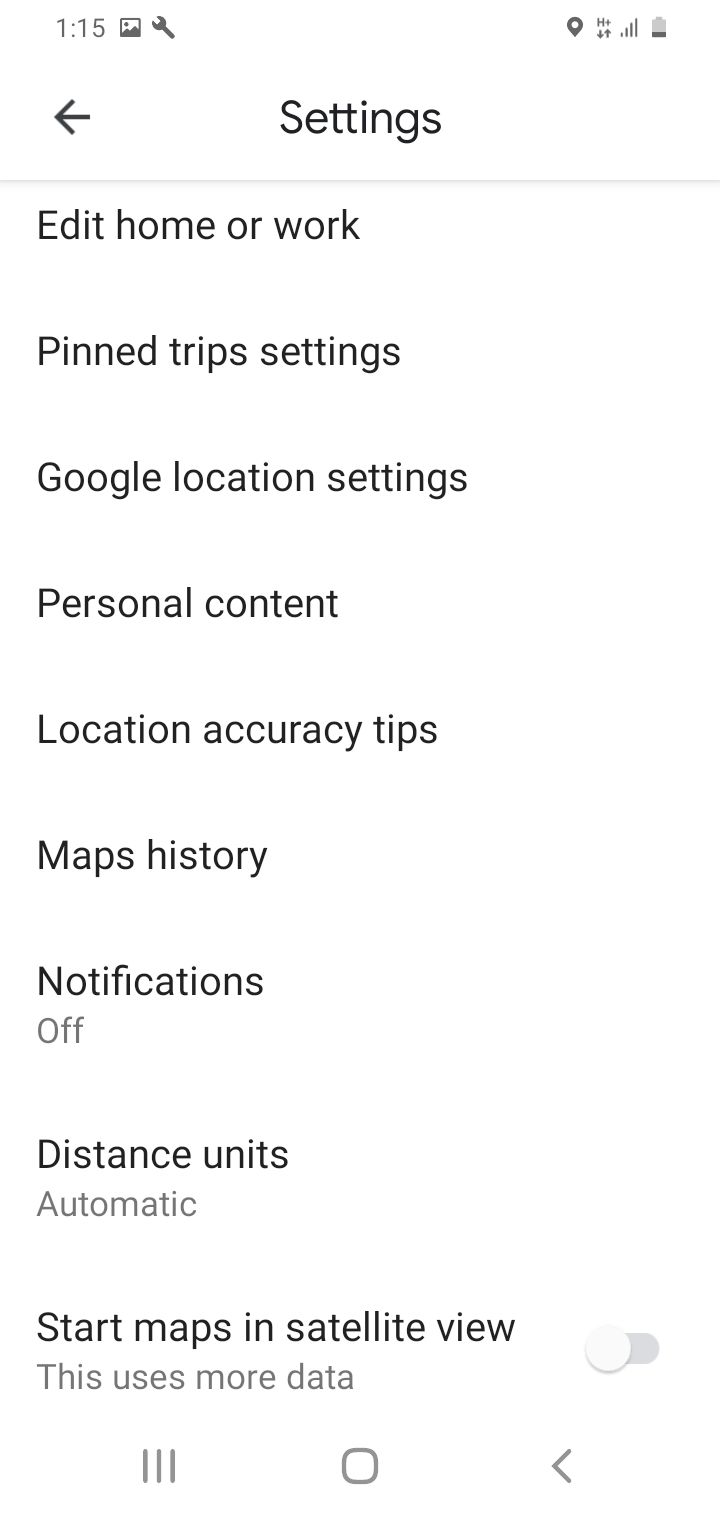This is a detailed screenshot of a mobile device’s settings page, captured in landscape orientation at 1:15 PM. The interface displays a white background with black text and various icons. Notably, there is a small wrench icon in the upper section, indicating that the user is currently modifying their settings.

Highlighted settings and features include:
- Location data: Enabled
- Hotspot: Enabled
- Signal strength: Full bars
- Battery level: Critically low at 20%
- Notifications: Disabled
- Distance units: Automatic
- Start maps in satellite view: Enabled (with a notice that it uses more data)

Specific visible options in the settings menu are as follows:
- "Edit home or work"
- "Pin to trip settings"
- "Google location settings"
- "Personal content"
- "Location accuracy tips"
- "Maps history"

The navigation buttons at the bottom of the screen are arranged as: 
- Context Button (left)
- Home Button (middle)
- Back Button (right)

This screenshot encapsulates key elements of the device's settings page, emphasizing location services, personalized settings, and noteworthy status indicators such as battery life and connectivity features.